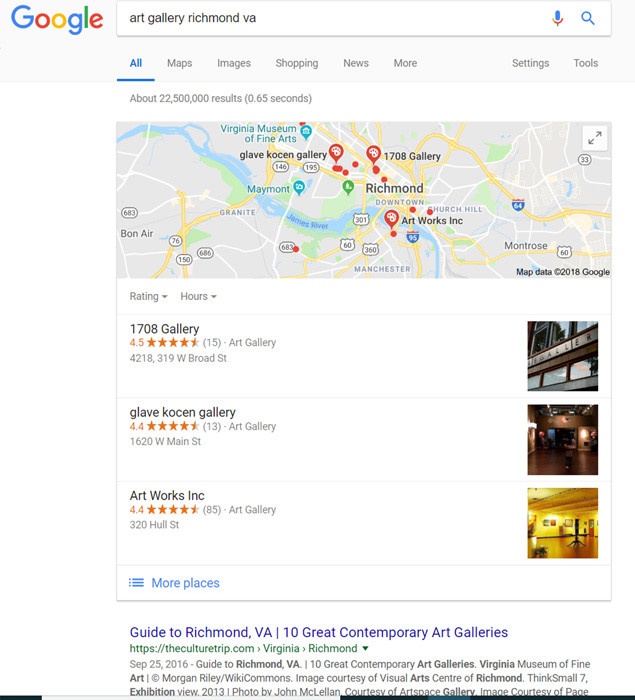This screenshot captures a Google search page for "Art Gallery, Richmond, Virginia." The user is currently on the "All" tab but has options to switch to "Maps," "Images," "Shopping," "News," "More," "Settings," and "Tools." The search yields approximately 22,500,000 results in 0.65 seconds. The page includes a map with 2018 Google data displaying various art gallery locations in Richmond, alongside a section devoted to ratings and operating hours.

Presently highlighted are three art galleries:
1. **1708 Gallery** - Located at 319 West Broad Street, it boasts a 4.5-star rating based on 15 reviews.
2. **Glaive Cosen Gallery** - Situated at 1620 West Main Street, it has garnered a 4.4-star rating from 13 reviews.
3. **Artworks, Inc.** - Found at 320 Hull Street, it holds a 4.4-star rating with 85 reviews.

Additionally, a featured search result from theculturetrip.com offers a guide titled "Guide to Richmond, Virginia: 10 Great Contemporary Art Galleries," providing further insights into the art scene in Richmond.